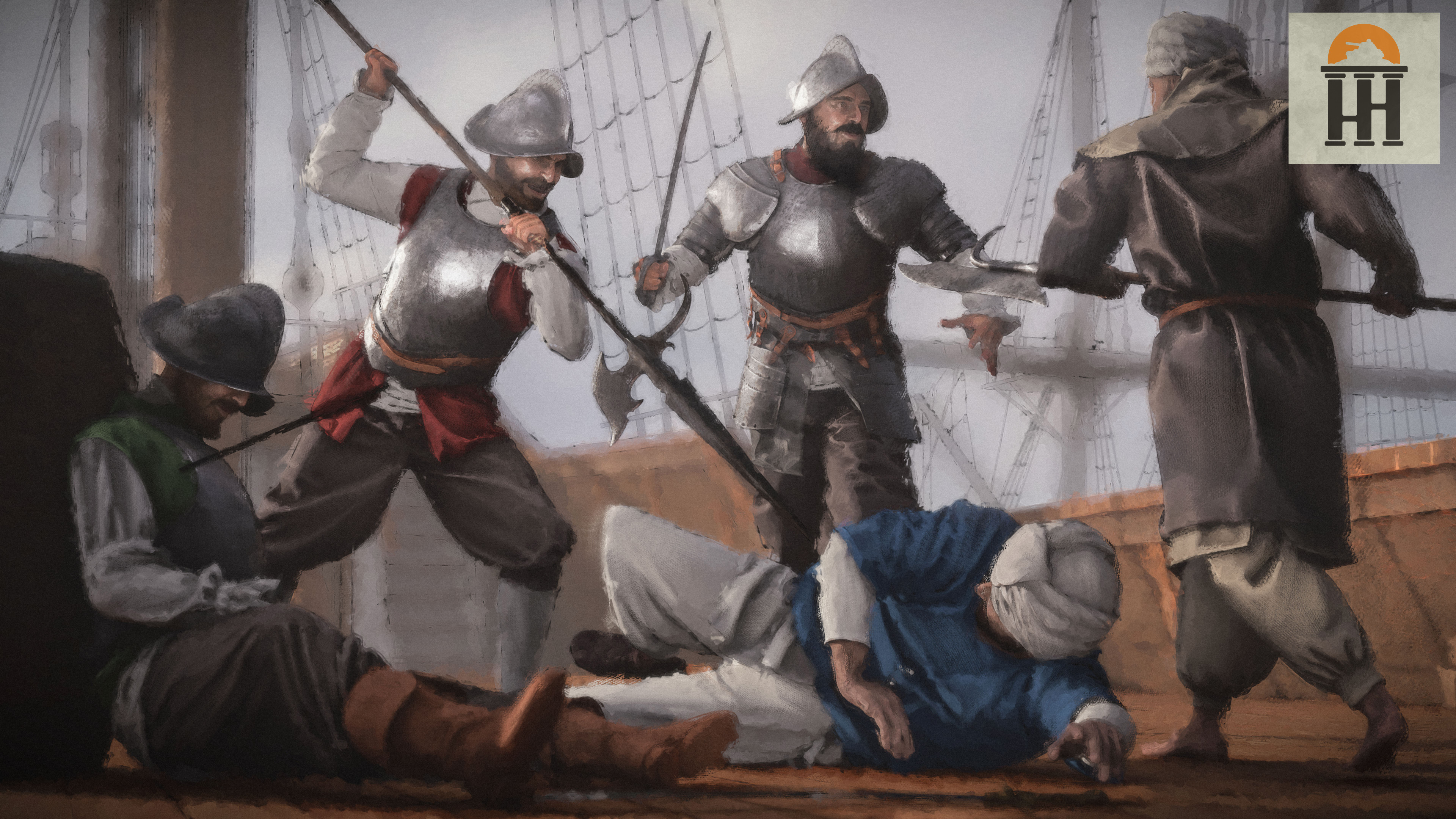The oil painting vividly depicts a chaotic battle scene set on the deck of a ship, potentially a pirate or conquistador raid given the maritime elements such as sails, ropes, and netting in the background. On the right side of the composition, a man in full armor with a distinctive conical helmet and chest plate is forcibly holding another man on the ground. This prone figure wears a white turban and a blue shirt paired with white pants, and he appears to be in grave danger, unable to rise as the armored man menacingly points a long spear at him.

Nearby, another armored figure, also clad in metallic gear including a helmet and breastplate, is engaged in a sword fight with an opponent wielding a hatchet-like weapon. This combatant in fuller armor confronts his foe with a sword while simultaneously bracing against the chaotic surroundings.

To the left, a tragic scene unfolds with a man slumped and lifeless, leaning against a chair with an arrow piercing through his chest from the right side. His helmet, fallen over his eyes, signifies his demise. The painting conveys a brutal and intense struggle, marked by the contrasting garments and weapons of the combatants. In the upper right corner, a small logo, 'HH,' can be seen, possibly the artist's signature or mark.